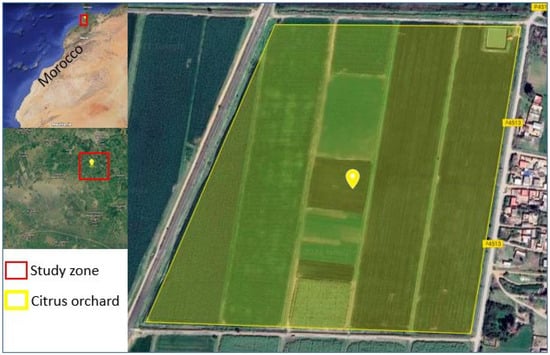The image features a detailed top-down satellite view of an agricultural area in Morocco, primarily showcasing a citrus orchard. The main section, making up about 85% of the image, highlights the orchard, sectioned off in a yellow grid, situated amidst surrounding farmlands with town buildings visible to the right. A small yellow tab marks the center of the orchard area.

On the left side, an inset map in blue and tan hues shows the broader location of Morocco, specifically highlighting the northwestern coastal region. Below this, a more zoomed-in view presents a red box outlining the study zone within the geographic area. An even closer view of this red-boxed study zone is provided at the lower part of the left-side insets.

A legend clarifies the color-coded sections: the red box denotes the study zone, and the yellow box indicates the citrus orchard. The layout of the image provides a comprehensive view, with a mix of dark and light green shades representing the landscape, alongside patterns denoting buildings on the sides.